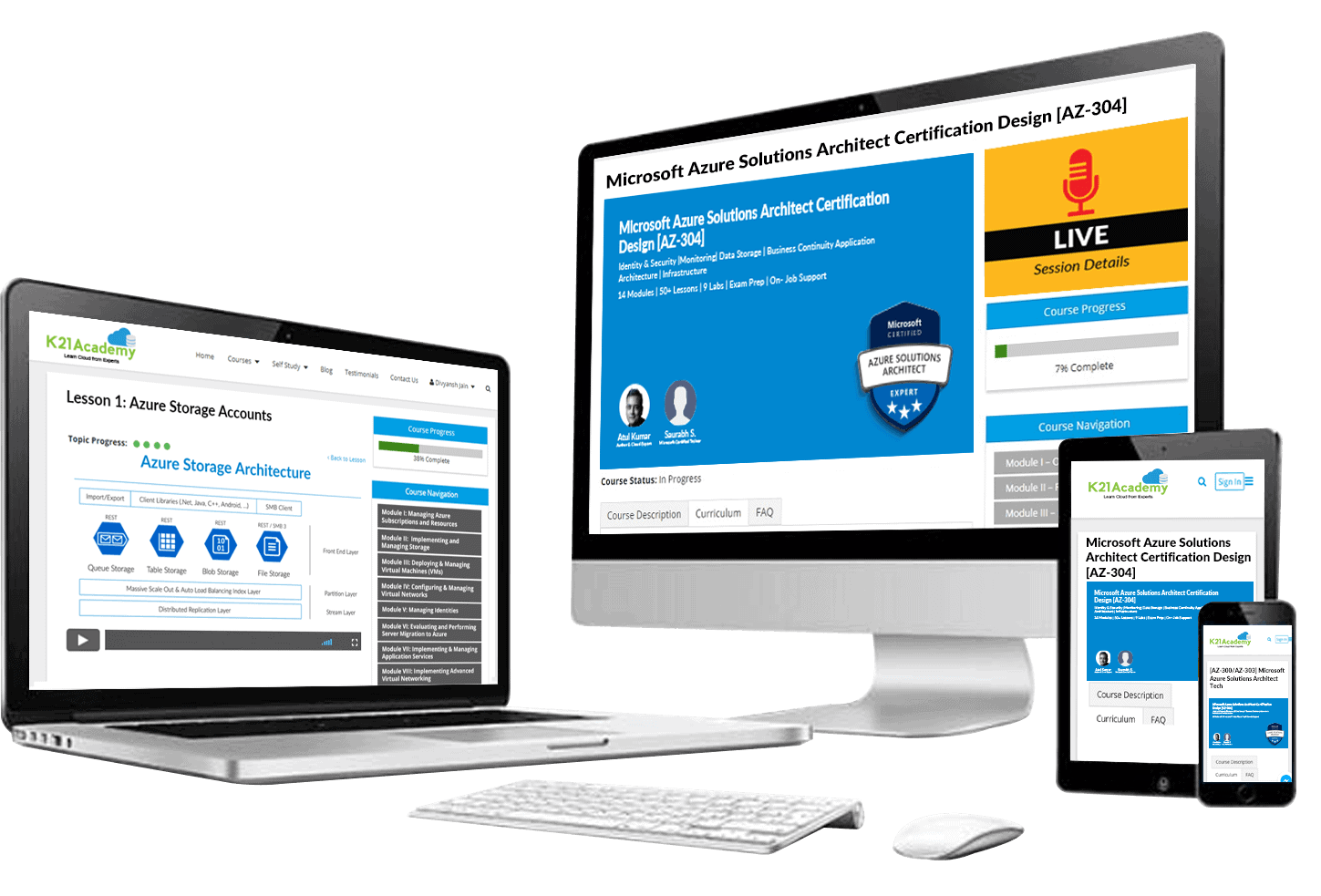The image depicts an advertisement for a website accessible on multiple platforms, set against a clean white background. On the left side, there is a sleek silver laptop with an open screen featuring a black border, silver base, and silver touchpad. The laptop has black keys and visible ports on the left side, potentially for an SD card, speaker, and charger. The laptop screen displays the K21 Academy website, identifiable by its green logo in the upper left corner. The website page shown is focused on "Lesson 1 Azure Storage Accounts," featuring a section titled "Four Stars Azure Storage Architecture" in blue, accompanied by four blue icons.

Positioned to the right of the laptop is a white wireless keyboard and a matching white wireless mouse, presumably for use with the Apple computer monitor in front of them. This Apple monitor has a sleek design with a silver curved base, a silver bottom frame, and a black frame around the screen. The monitor displays a white-background page with black text reading "Microsoft Azure Solutions Architect Certification Design (AZ304)" at the top, along with a blue square containing the same certification title. Below this section, there are two circles with faces or silhouettes and names underneath, followed by a badge labeled "Microsoft Azure Solutions Architect Expert" with three stars. Further to the right on the monitor, there is a yellow box with a red microphone icon and a black box with white text that says "LIVE SESSION" in capital letters. The session details list the progress of Azure completion at 7%, displayed with a green progress bar.

On the right side of the image, there is a black iPad and a black iPhone, both showing the same screen as the Apple monitor. The iPad and iPhone screens feature the K21 Academy logo and the Microsoft Azure Solutions Architect Certification Design page.

The entire setup suggests a seamless integration of the K21 Academy website across various devices, highlighting the availability of their courses on laptops, Apple desktops, tablets, and smartphones.